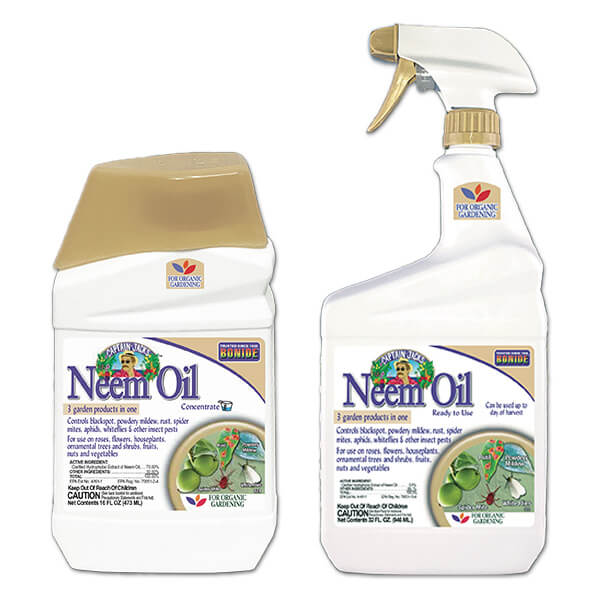Here is the revised and detailed caption:

---

This image showcases two organic gardening products, packaged in predominantly white containers with gold accents. The labels are white, featuring a prominent graphic at the top depicting a man wearing sunglasses, a hat, and a pink shirt, surrounded by various plants. Below the graphic, the product name "Neem Oil" is printed in a navy font, along with the phrase "Three garden products in one," also in navy. Additional information in navy and black font, including caution warnings, is provided at the bottom of the labels. The detailed graphics on the lower part of each container illustrate insects, green plants, and vibrant red flowers. Notably, one container is a spray bottle, while the other has a tan-colored lid, making them both visually distinct yet cohesive in design.

---

I hope this meets your needs! Feel free to ask if you need further tweaking!